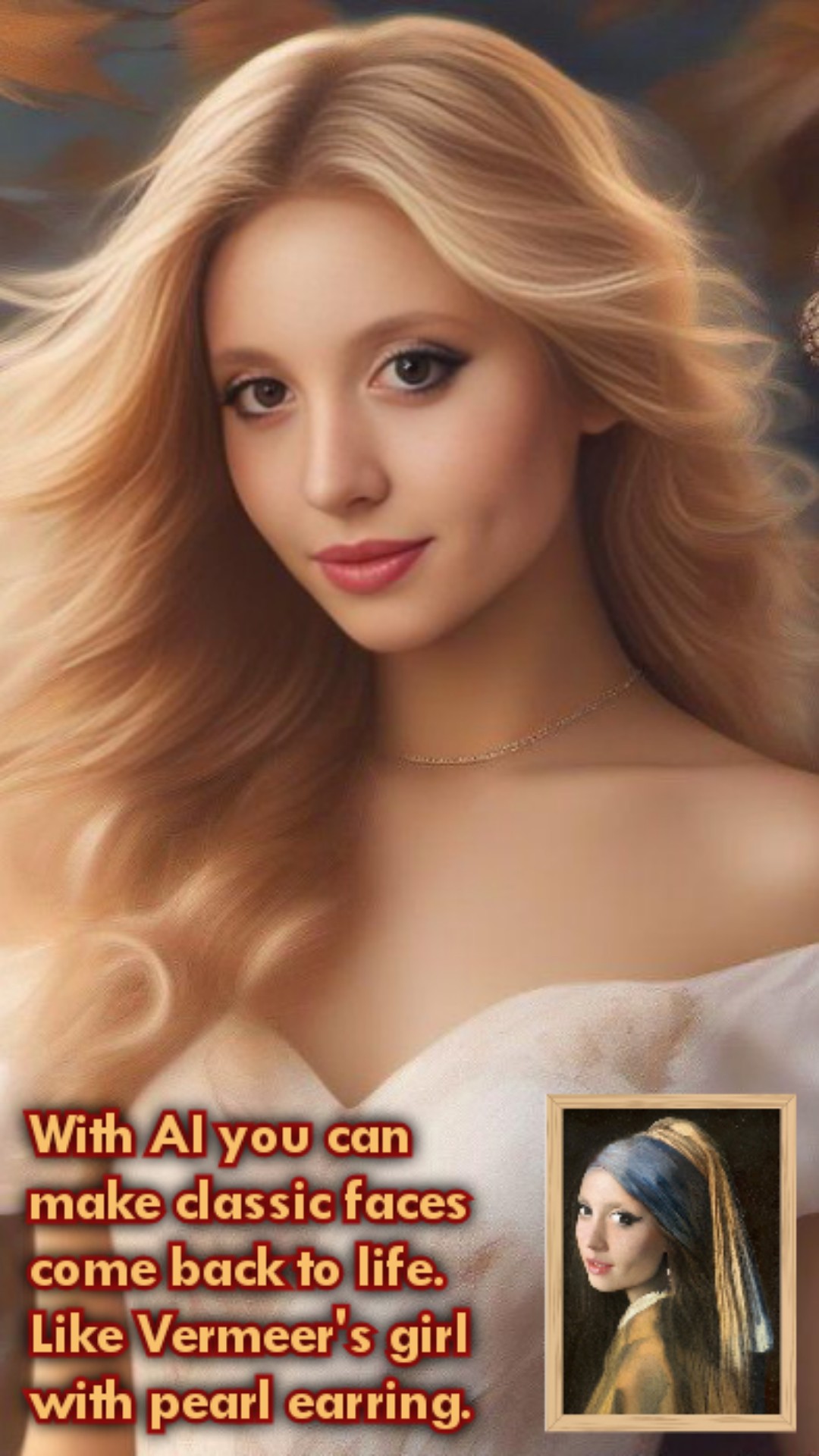This image features a computer-generated, realistic-looking young woman with blonde hair that flows gracefully around her pale face. Her dark eyes and pink lips stand out against the soft movement of her hair. She is adorned with a gold chain around her neck and wears a strapless, white gown with a cut neckline. The background is a warm brown, contrasting with her light complexion. 

In the lower left corner, text reads, "With AI, you can make classic faces come back to life, like Vermeer's Girl with a Pearl Earring." In the lower right corner, there is an inset frame, outlined in gold, showing a painting of another young woman. This inset figure, presented from the shoulders up, has a striking resemblance to the main image but is depicted with dark hair, a gold scarf on her head, and a gold-colored shirt. She is slightly turned to the left, looking towards the viewer, echoing the classic pose from Vermeer’s famous painting. Both figures highlight the transformative power of AI in recreating historic artworks with lifelike detail.